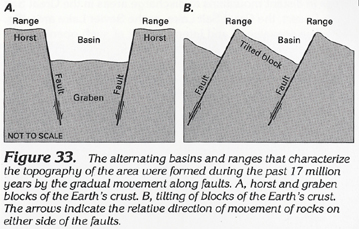The image is a detailed graphical illustration from a geology textbook, labeled as Figure 33, that explains the formation of topographic features over the past 17 million years through gradual fault movements. The illustration is divided into two parts, marked A and B, both presented in black, white, and grayscale.

Figure A depicts the Horst and Graben blocks of the Earth's crust, with labeled elements including "Range," "Horst," "Basin," "Fault," and "Graben." In this diagram, the Horst (elevated block) and Range are shown at the top, while the Basin forms a flat area below them, and the Fault and Graben (lowered block) are positioned beneath the Basin. The faults in this section are curved inwards towards each other.

Figure B illustrates the tilting of crustal blocks, featuring labeled components like "Fault," "Range," "Tilted Block," and "Basin." Here, the faults are parallel rather than curved, and the tilted block creates a V-shaped basin.

Both sub-figures include arrows indicating the relative direction of rock movement along the faults. The entire graphic is identified as not to scale, emphasizing that it is a conceptual representation rather than an accurate geometric model.